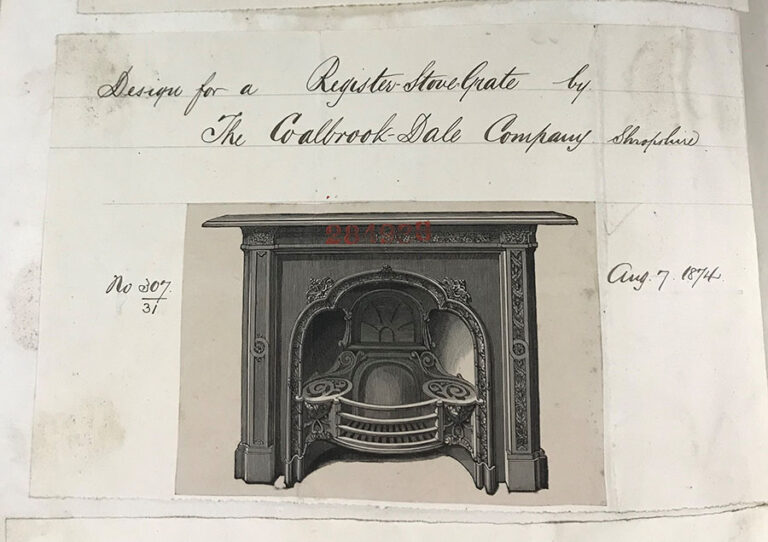The image depicts a detailed, hand-drawn illustration of a fireplace and register stove grate by the Colebrookdale Company, dated August 7, 1874. The artwork, rendered in dark gray colored pencil on off-white paper, showcases a fireplace with an ornately carved mantle and a grate featuring four metal bars and side plates, potentially for cooking. Above the image, a caption in elegant cursive script reads, "Designed for a Register Stove Grate by the Colebrookdale Company." The number 207 is noted to the left of the fireplace, indicating its position in what appears to be an old advertisement booklet or a page from a historical design catalog, suggesting it was perhaps copied to enhance clarity.